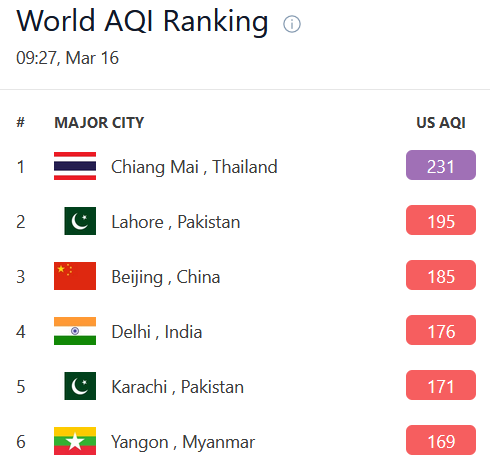**World AQI Ranking**

This image shows the World AQI (Air Quality Index) Ranking with a clean, white background and black text. In the upper left corner, in bold, it reads "World AQI Ranking," next to a gray circle with a white interior containing a lowercase "i." Directly below this, it displays "0927, March 16th" on the left side, followed by a thin, horizontal gray line.

Below the line, the list begins with a header row that features a number sign "#" followed by "Major City." The rankings are as follows:

1. **Chiang Mai, Thailand**: Accompanied by an outline of a Thai map on the left and the label "US AQI" on the right, it is highlighted with a purple rectangle containing the number "231" in white text.
2. **Lahore, Pakistan**: Marked by a Pakistani flag, the city is listed with a red rectangle displaying the number "195."
3. **Beijing, China**: Featuring a Chinese flag, the listing is highlighted with a red rectangle indicating the number "185."
4. **Delhi, India**: Illustrated with an Indian flag, it follows a red rectangle showing "176."
5. **Karachi, Pakistan**: With a Pakistani flag, the city is followed by a rectangle marked "171."
6. **Yangon, Myanmar**: Displayed alongside a Myanmar flag, the city's AQI is presented in a rectangle with the number "169."

The image provides a clear and detailed visual representation of the global air quality rankings, prioritizing both aesthetic simplicity and informative value.